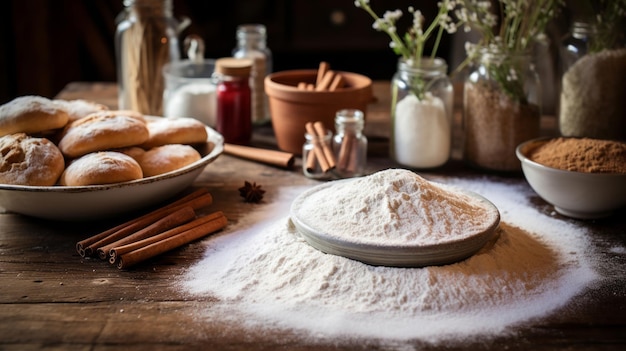This editorial-style photograph showcases a rustic wooden table adorned with various baking ingredients, meticulously arranged to evoke a sense of warm, homely preparation. Central to the image are several key elements: a white bowl overflowing with flour, surrounded by a fine dusting of sugar, which creates a textured contrast on the table. Additional bowls contain brown sugar and what might be more ground cinnamon or another brown spice. There's a collection of jars, each filled with different powders, spices, and possibly seeds or legumes, contributing to the rich mosaic of textures and colors. Cinnamon sticks are prominently featured both in a terracotta pot and scattered directly on the table, while a bowl of freshly baked rolls sits invitingly off to the side, presumably the result of these very ingredients. Decorative plants in jars add a touch of greenery in the background, enhancing the image's aesthetic appeal without overpowering the primary focus on the baking essentials. This vivid and intentional arrangement makes the photograph ideal for a blog or magazine spread on baking or rustic kitchen charm.